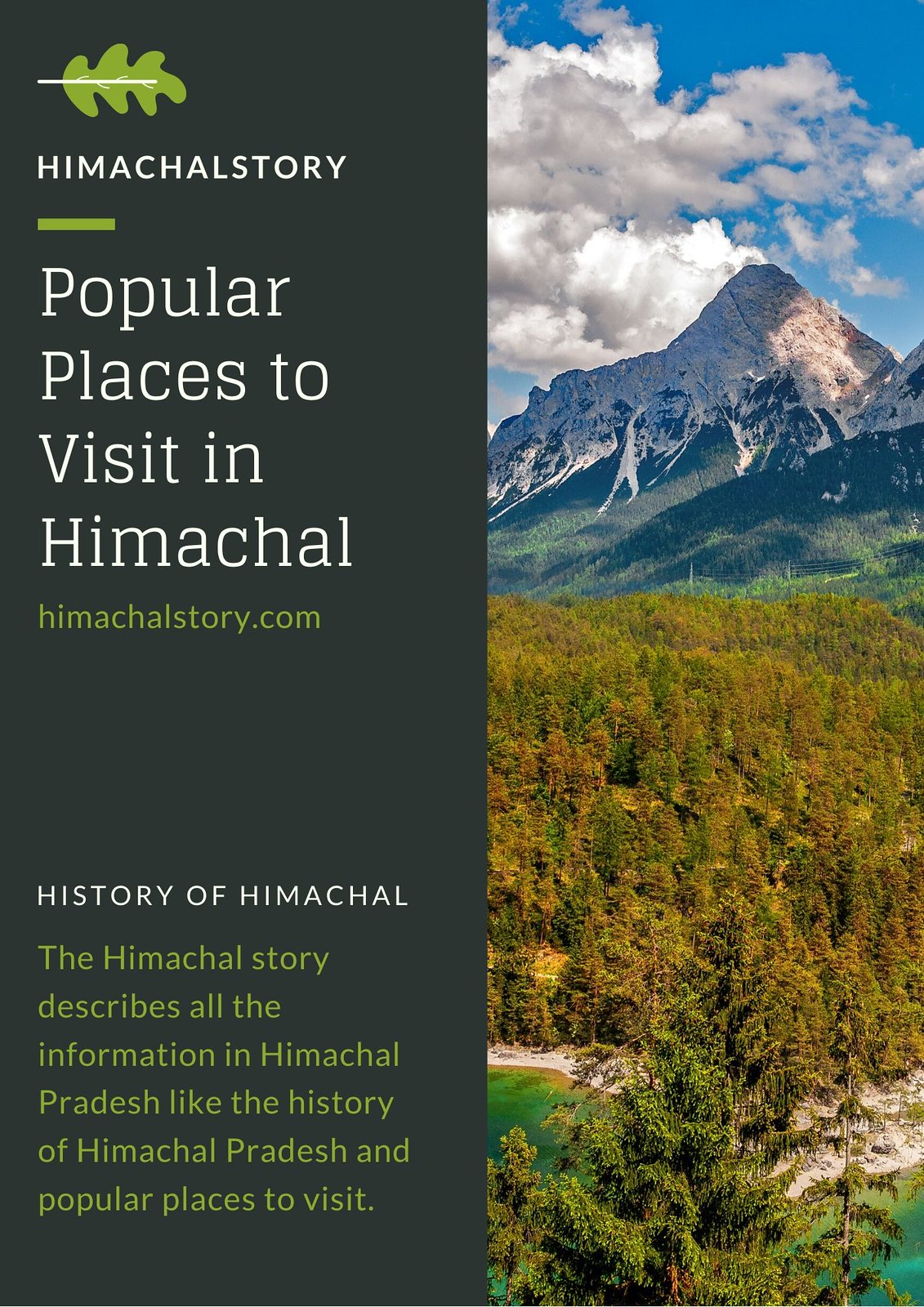The poster features a vertically divided design. On the right half, a stunning nature photograph captures a breathtaking mountain range under a blue sky dotted with fluffy white clouds. Below the mountains, dense green shrubbery and numerous trees dominate the middle ground, while a small body of water lies in the lower corners.

The left half of the poster is a gray panel filled with informational text in white and green. At the top, an illustration of a three-pronged leaf is followed by the title "Himachal Story." Below it, in bold white print, it reads, "Popular Places to Visit in Himachal." Further down, in green text, it lists "HimachalStory.com." Near the bottom left, in white text, "History of Himachal" appears, followed by a green description that states, "The Himachal story describes all the information in Himachal Pradesh, like the history of Himachal Pradesh and popular places to visit."